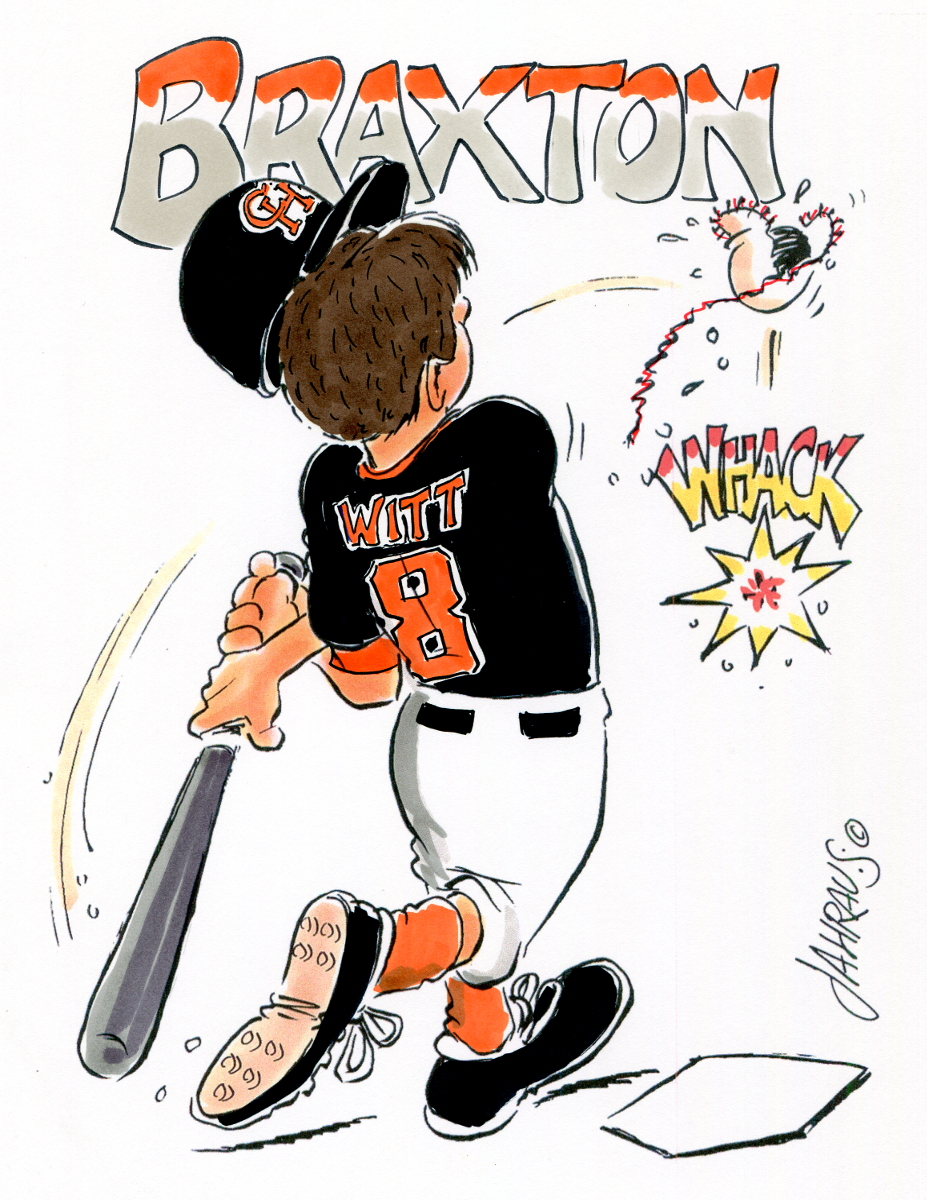In this detailed image, we see an animated scene featuring a boy playing baseball. Dominating the top portion of the image is the name "Braxton," prominently written in all uppercase, bubble letters with a color gradient from orange at the top to gray at the bottom. The scene captures the boy mid-swing, just after hitting a baseball. The baseball has been dramatically split open from the force, revealing a black interior with red stitching unraveling around it. A vibrant "Whack" on the right side, depicted in a mix of red, white, and yellow along with a starburst effect, accentuates the impact of the hit.

The boy is dressed in a typical baseball uniform. He wears a black and orange hat emblazoned with the initials "CH" in orange, outlined in white. His jersey, primarily black with orange accents, bears the name "WIT" and the number "8" on the back. He pairs his jersey with white baseball pants secured with a black belt, tucking his orange socks into his black-and-orange shoes that are orange at the bottom and black along the sides. The boy's gray bat is frozen in action as he stands over a white home plate base, marked by his determined stance and swinging motion.